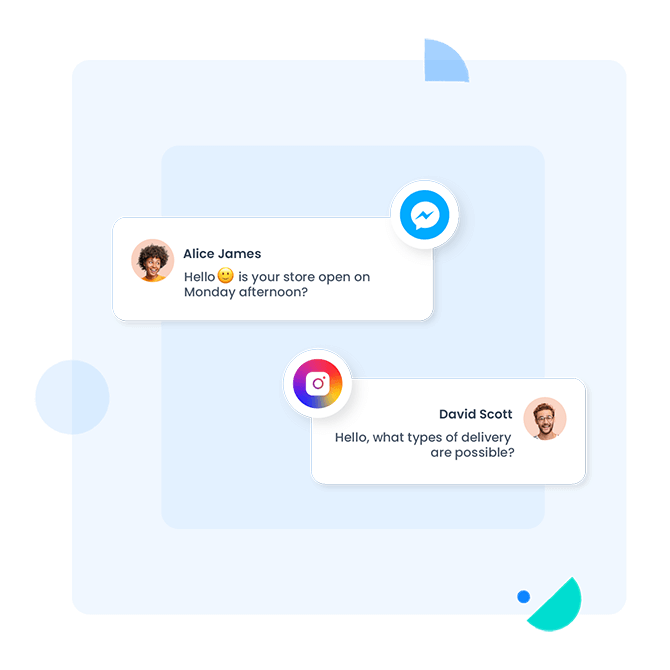A screenshot showing a chat interface between two individuals, Alice James and David Scott. On the middle-left side of the image, there's a rectangular chat box. Inside this box, on the far left, is a profile picture—a circular image featuring a black woman with an Afro hairstyle, warmly smiling and looking to the right. Her face is visible down to the neckline. To the right of this image, the name "Alice James" is displayed, followed by her message that reads, "Hello😊? Is your store open on Monday afternoon?" At the top right corner of this chat box is a small blue circle with a sideways lightning bolt icon.

Directly below this, on the bottom right, there's another rectangular chat box. This time, the profile picture is on the far right, depicting a white man with glasses, a beard, and short hair. To the left of his profile picture is the name "David Scott," accompanied by his message: "Hello, what type of deliveries are possible?" In the top-left corner of this chat box is an Instagram icon. The overall interface suggests a messaging application where users can engage in conversations with various individuals.